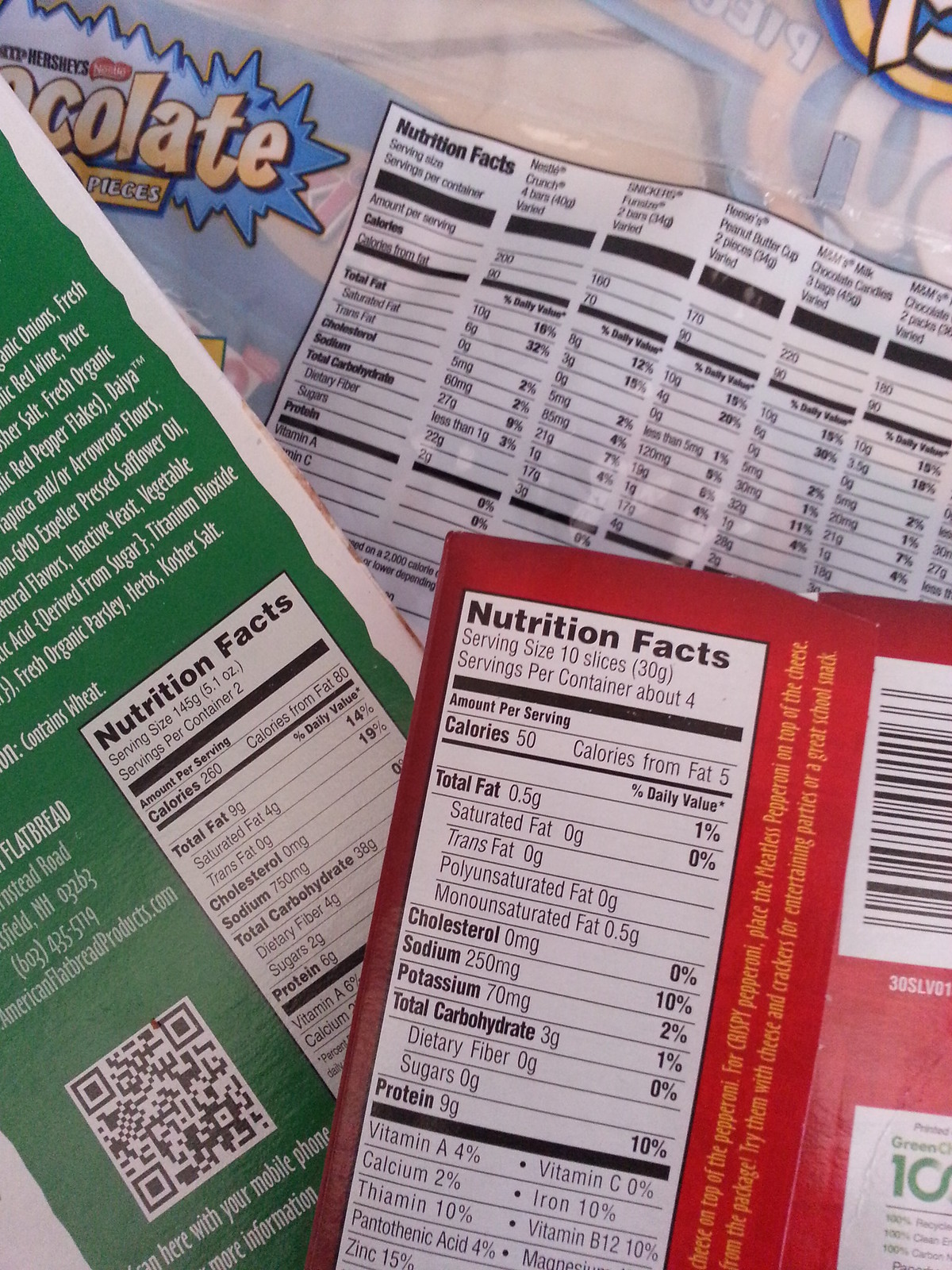This photograph features a cluttered arrangement of three different products, primarily displaying their nutritional facts. In the background, a partially visible plastic package reveals the word "chocolate" against what seems to be a blue, spiky bubble design, hinting at Nestle Crunch pieces bars, which detail 200 calories for four bars. In the foreground, a green package, likely for American flatbread, prominently displays its nutrition facts alongside a square QR code, noting 260 calories per 145 grams. Topping the pile, a flattened red cardboard box shows both its nutrition facts, specifying a serving size of 10 slices with 50 calories each, and a barcode, though the exact product remains unidentified. The overall scene gives a chaotic yet informative snapshot of the nutritional details of these snack items.